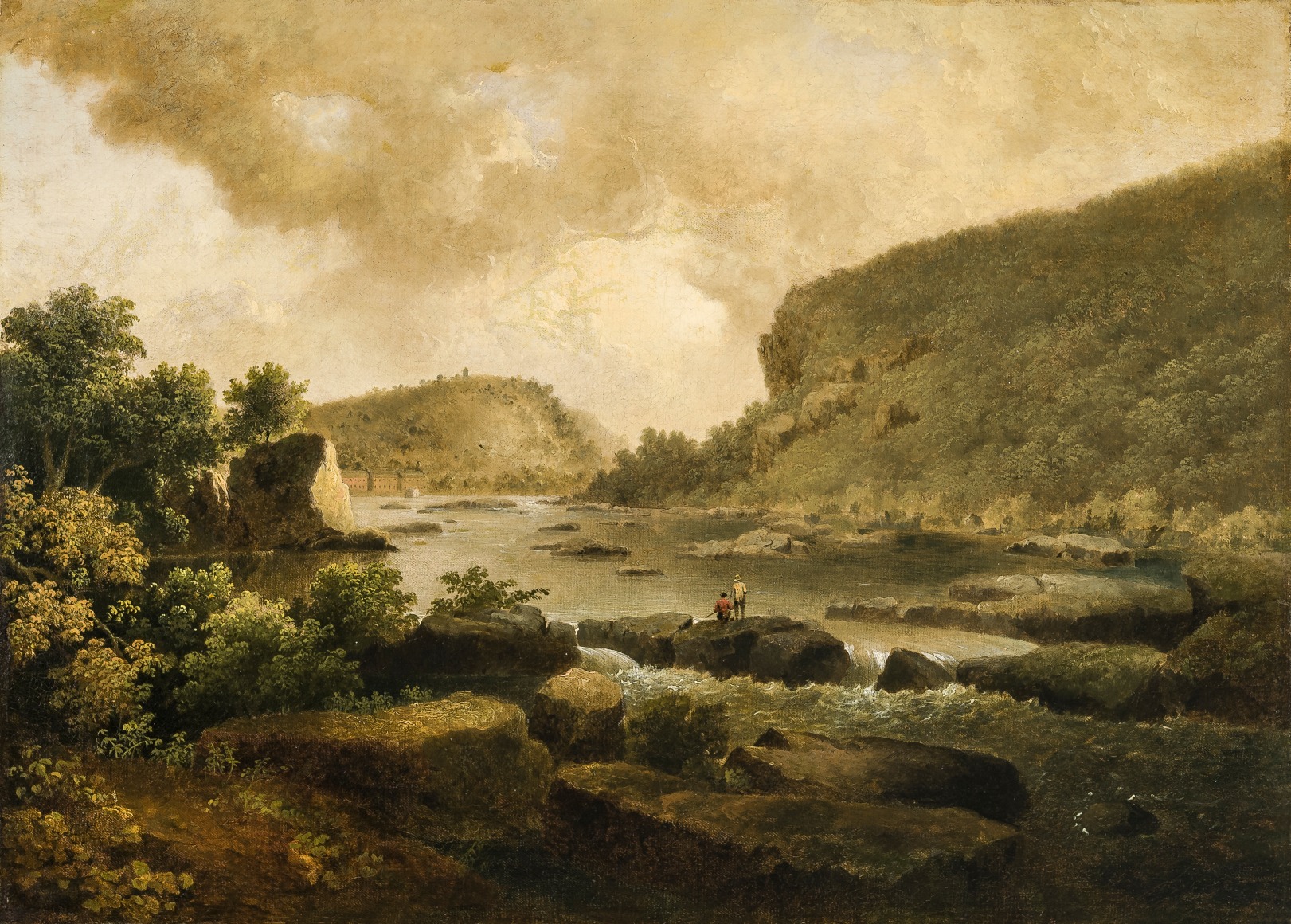The image depicts a warm, sepia-toned oil painting of an outdoor scene featuring a lake with a rocky stream running through it, surrounded by overgrown trees, bushes, and large rock formations. Two individuals are standing on the rocks near the water's edge, either looking out onto the lake or possibly engaged in fishing; one is wearing a red shirt, while the other is dressed in a white or yellow shirt with a large-brimmed hat, possibly a cowboy hat. The colors in the painting are predominantly warm tones of brown, yellow, cream, with touches of green and rust, imparting a vintage feel to the scene. The surrounding landscape includes what appear to be small islands or hills near the water, with dense plant life throughout. The sky is overcast and cloudy, contributing to the overall warm yet subdued atmosphere of the painting. In the background, large hills covered with trees and brush rise behind three brick houses, enhancing the scenic and rustic quality of the image.